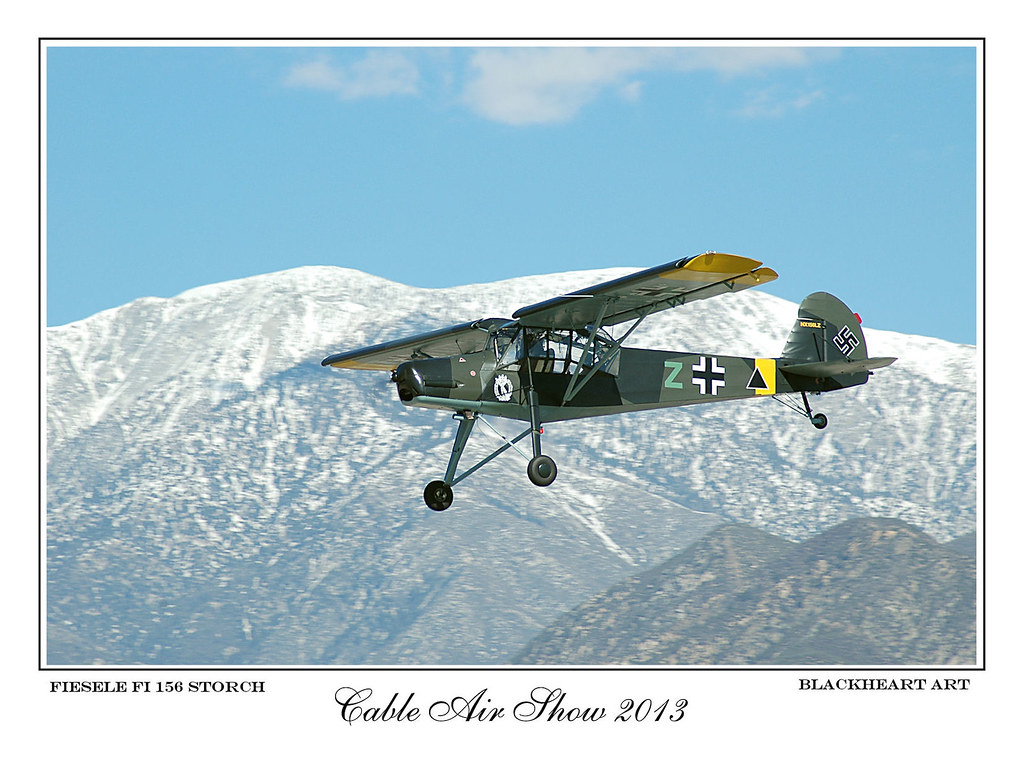This captivating image, captured during the Cable Air Show in 2013, portrays a distinctive camouflage-green biplane in mid-flight, soaring amidst the snowy peaks of large mountains under a light blue, cloud-speckled sky. The biplane, which appears centrally in the photograph and oriented towards the left of the frame, features various markings and symbols. These include a prominent black swastika on the tail, a white and black cross, a black triangle with a yellow rectangle, and a green 'Z'. The rugged mountains in the background display a mix of snow-covered summits and brown, snow-scattered lower sections. The scene is set against a backdrop of crisp Snow White, Sky Blue, Army Green, Yellow, Black, White, Light Green, and Red hues, all contributing to the vivid winter landscape and the historical aviation theme. This image, curated by Blackheart Art, also bears text labels reading "Pearson, Florida, 156 Storch, Cable Air Show 2013".